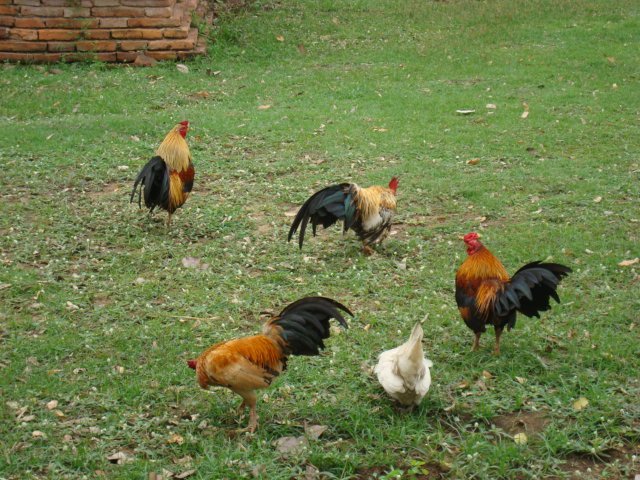This color snapshot captures a vibrant backyard scene with five chickens, four of which resemble roosters, and one white chicken pecking at the ground. The roosters, which may actually include hens given their number, exhibit striking dark reddish-brown feathers with long, iridescent greenish-black tail plumes. The birds also display the common red combs and wattles characteristic of roosters. The grassy lawn is dotted with fallen leaves, adding a touch of autumnal charm. In the upper left corner of the image, there are several layers of aged, multicolored bricks forming a corner structure—potentially the base of a chimney or a wall fragment. The white chicken in the foreground, with her rear end elevated as she pecks in the dirt, adds a playful touch to the pastoral scene.